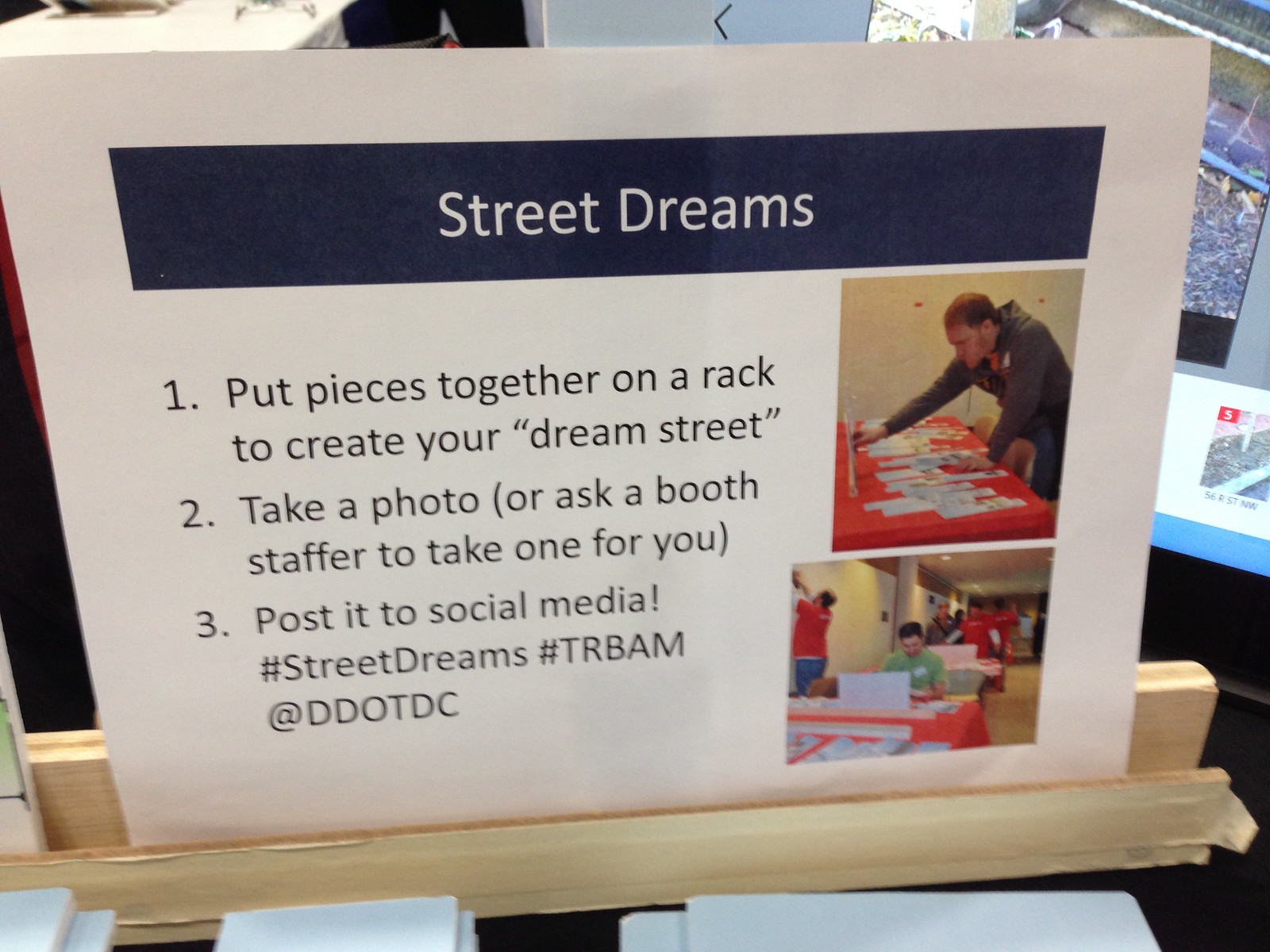The image captures a detailed poster titled "Street Dreams," displayed on a wooden board apparatus designed to hold pictures or documents. The background of the poster is white, with a black bar at the top featuring the title. The poster includes two images and instructions in black text. Listed beneath the title are three bullet points labeled 1, 2, and 3. 

The first image, located on the left side of the poster, shows a man leaning over a table, working with various objects to create a display. The second image, to the right, appears to show another man either working on a laptop or designing his dream street setup, though it's likely the latter based on the context.

The instructions read:
1. Put pieces together on a rack to create your dream street.
2. Take a photo or ask a booth staffer to take one for you.
3. Post it to social media with the hashtags #streetdreams, #trbam, and tag @ddotdc.

Surrounding the poster, there seem to be people at a fair or event, possibly there to help participants with the activity. The wooden racks and various cards or objects mentioned in the instructions are laid out on the table beneath the poster, inviting attendees to engage in the creative process and share their work online.